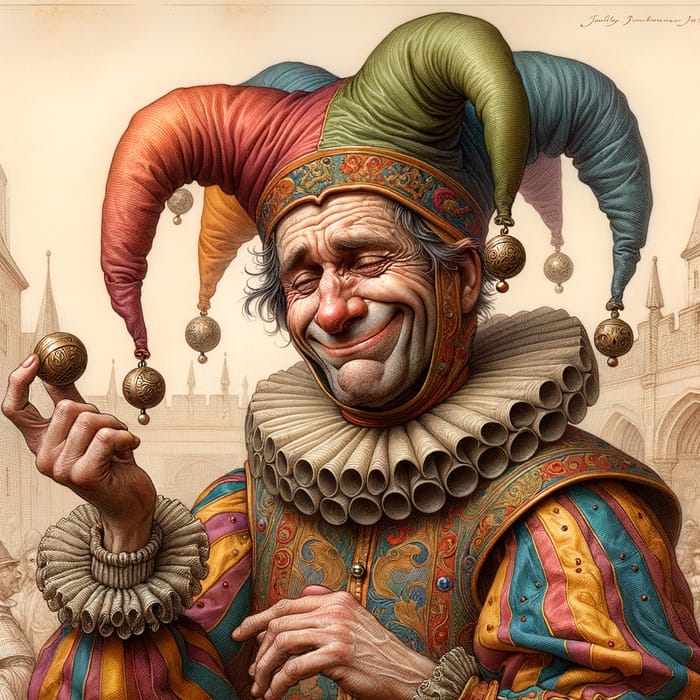This is a detailed drawing of an elderly Caucasian court jester, shown from mid-chest upwards. The artwork measures approximately 5 inches square, with a background featuring faded brown buildings and people in a courtyard, creating a somber atmosphere beneath an off-white brown sky. 

The jester is adorned in a vividly colored outfit: a shirt with vertical stripes of red, yellow, and blue, and a similarly ornate vest with intricate red and blue paisley-like patterns. His face is wrinkled with grayish-black hair, and his red lips form a smile that hints at a mixture of joy and melancholy.

His distinct five-pointed hat stands out with its blue, red, green, yellow, and orange sections, each decorated with a gold bell at the tip. The hat's band drapes beneath his chin, and his eyes are closed as he slightly faces left. Surrounding his neck and wrists are large, spiraled white and off-white ruffles that match, adding to the whimsical yet detailed portrayal. His right hand is raised, holding a small gold ball resembling a Christmas ornament, while his left hand is positioned in front of him. 

A signature is present in the upper right corner, though it is illegible. The image captures the essence of the jester in elaborate detail, emphasizing the textures and colors that bring this character to life.